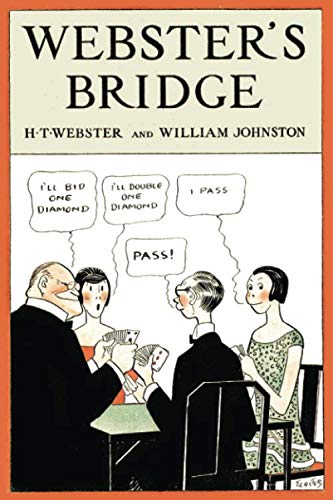The cover of the book Webster's Bridge, illustrated with an orange border and a light tan background in the upper third, features black text in a large sans-serif font reading "WEBSTER'S BRIDGE" at the top. Below the title, in smaller text, are the authors' names: H. T. Webster and William Johnston. The main image occupying the bottom two-thirds displays a well-designed cartoon drawing of a card game. Four people—two men and two women—are seated around a square poker table, all holding cards. Both men are in tuxedos, with the man on the left facing the viewer, saying, "I'll bid one diamond." To his left, a woman in a red dress responds, "I'll double one diamond." The second man, turned towards the others, declares "pass," followed by the woman on the far right in a green and white poker dress, who also says, "I pass." Each character’s dialogue is captured in speech bubbles above their heads, contributing to the engaging and meticulously crafted artistic design.